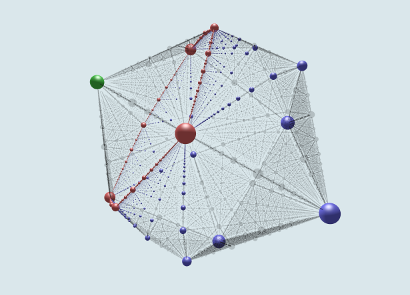This image depicts a three-dimensional structure resembling a hexagon or possibly an octagon, composed of numerous small, multicolored spheres connected by an intricate web of lines. At the center of the shape is a prominent red sphere, which serves as a focal point. Radiating from this central sphere are various lines linking it to other spheres of different sizes and colors, predominantly blue, red, and green. The spheres are organized in clusters based on their color, with blue, red, and green groups positioned strategically around the central red sphere. There are also transparent gray spheres interspersed throughout the structure, likely indicating points of depth or elements on the reverse side of the object. The entire assembly is set against a light blue background, which highlights the vivid colors and complex connectivity of the spheres and lines. The image appears to be a detailed mapping or network visualization, with each sphere and line possibly representing specific points and connections within a larger system.